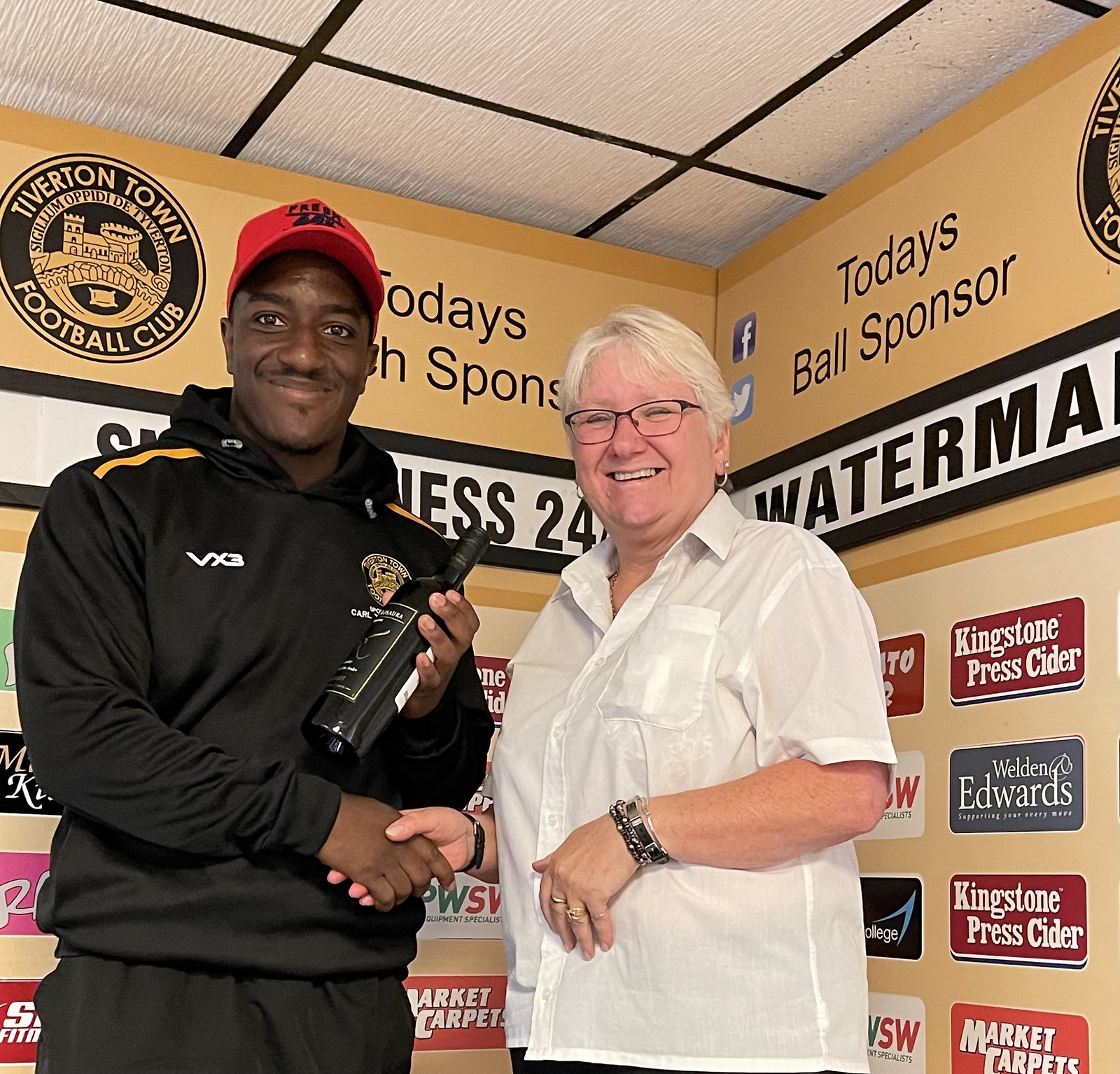In this photograph taken indoors, a black gentleman, seemingly in his 20s or 30s, stands on the left, dressed in black athletic clothing—a hoodie and sweatpants—topped with a red hat featuring black letters. His right hand is extended in a handshake with an elderly white-haired woman who appears to be in her 60s or 70s. She wears a white blouse, glasses, and wrist jewelry. The gentleman holds a bottle of wine in his left hand. They pose in front of a yellow wall adorned with various sponsor logos. Prominently displayed at the top is the Tiverton Town Football Club crest, depicting an old castle illustration. Below the crest, other sponsor names are visible, including Kingston Press Cider, Weldon Edwards, and Market Carpets.